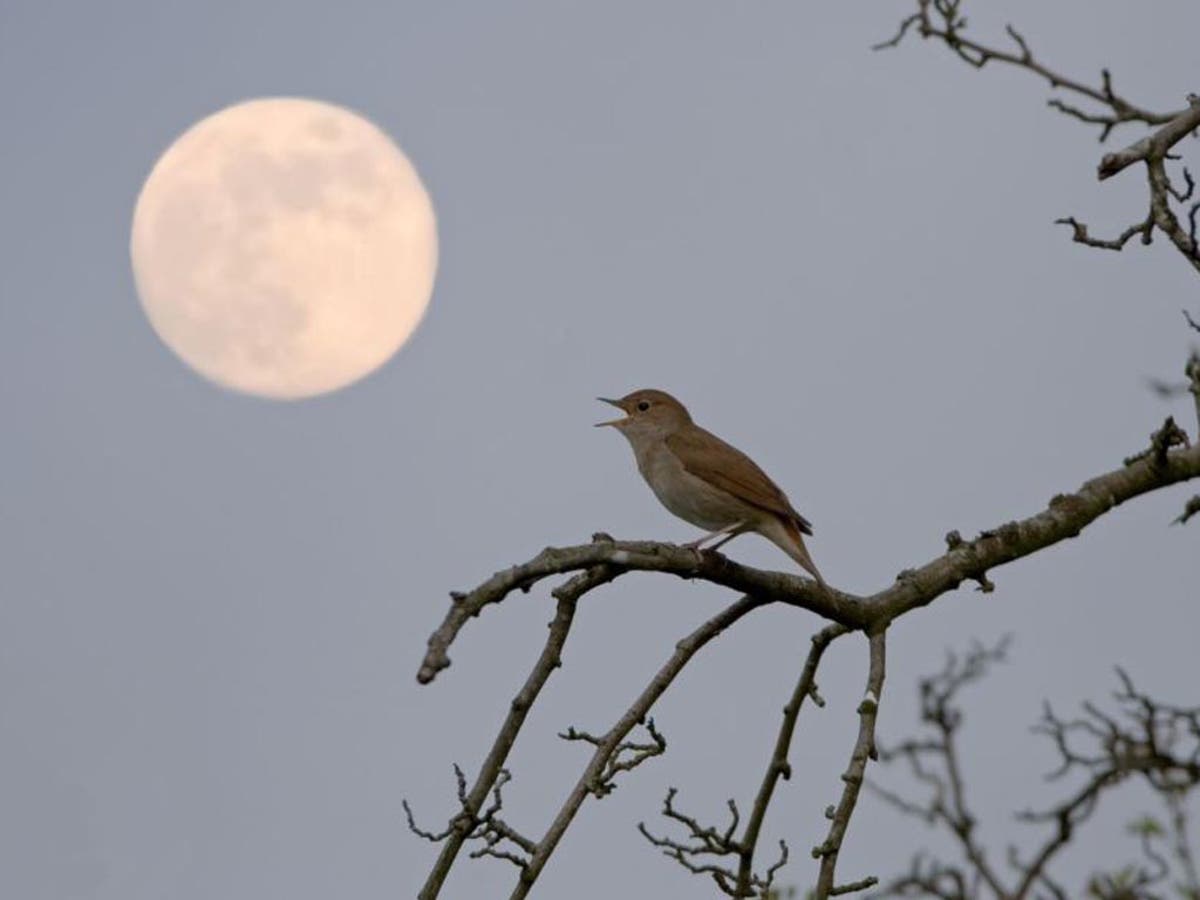In this outdoor night scene, a small sparrow with a brown wing, grayish underbelly, and dark brown head perches on a twisted, leafless branch that extends from the right into the center of the image. The bird, facing left with an open beak as if chirping, has a light brown belly and neck, light brown tail feathers, and little black beady eyes. The intricate branches supporting the bird are brown and gray, with thicker sections where the bird is perched. In the background, the sky transitions from blue to gray, revealing a large full moon in the top left corner, casting a dim light over the scene. The overall ambiance suggests late evening, with a serene yet slightly eerie quality, emphasized by the barren trees scattered in the distance.